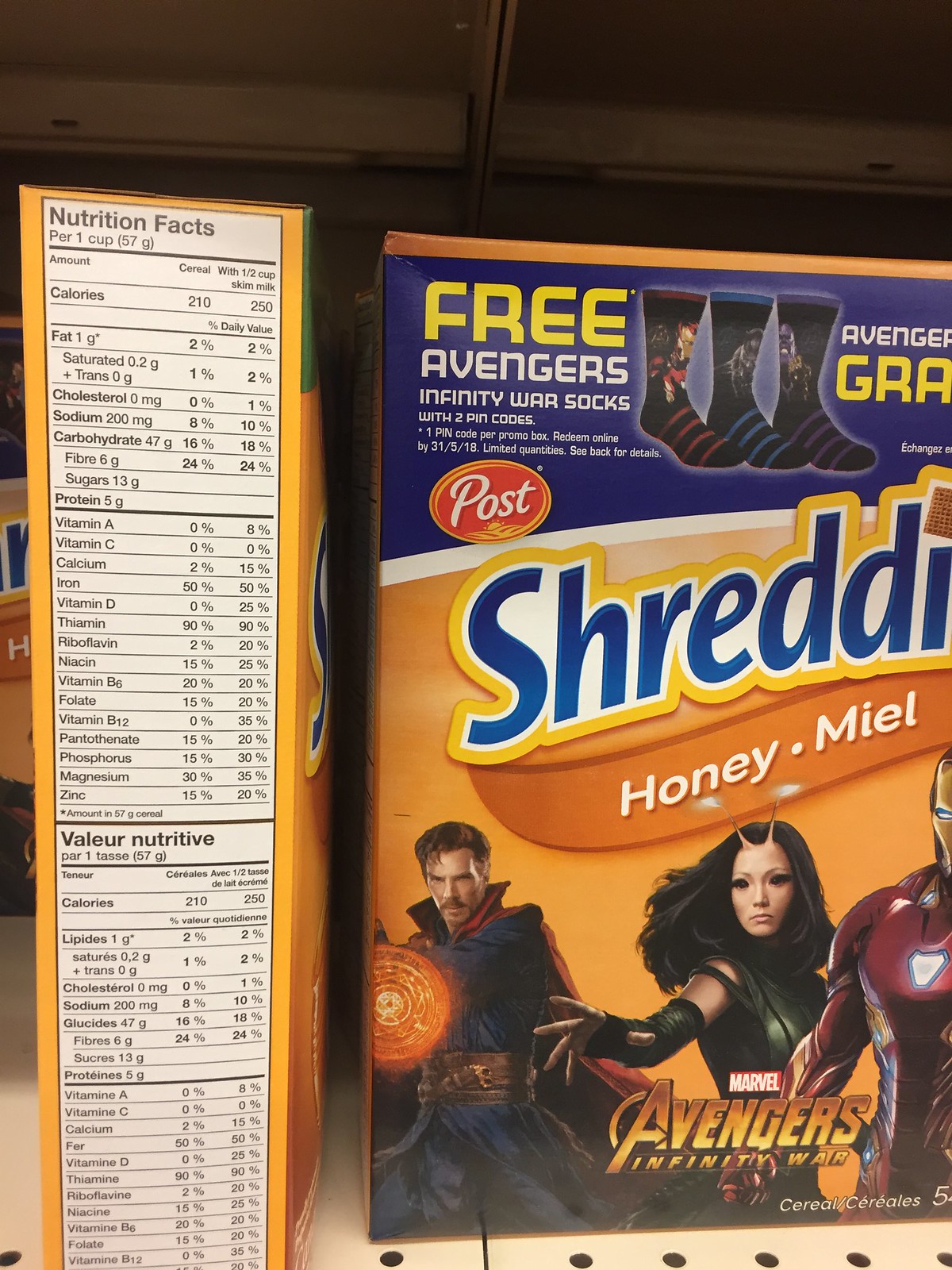The image depicts a cereal box prominently featuring an orange-themed design. The brand name "Post" is displayed at the top in white font set against a blue background. Below this, in a red background, the product name "Shredded Wheat" is visible. The text "Honey Miel" appears underneath the product name, accompanied by an orange swirl graphic.

The cereal box is shown from two perspectives: the front view on the right and the side view laying down on its left. Marvel characters are featured on the front of the box, including Doctor Strange, Iron Man, and another female character. Above the branding, there is a promotion for "Free Avengers Infinity War socks with two pin codes," illustrated with three sock designs next to the promotional text.

The side view of the box includes the nutrition facts panel set against a white background. Both boxes are displayed on a shelf, suggesting they are located in a retail setting.